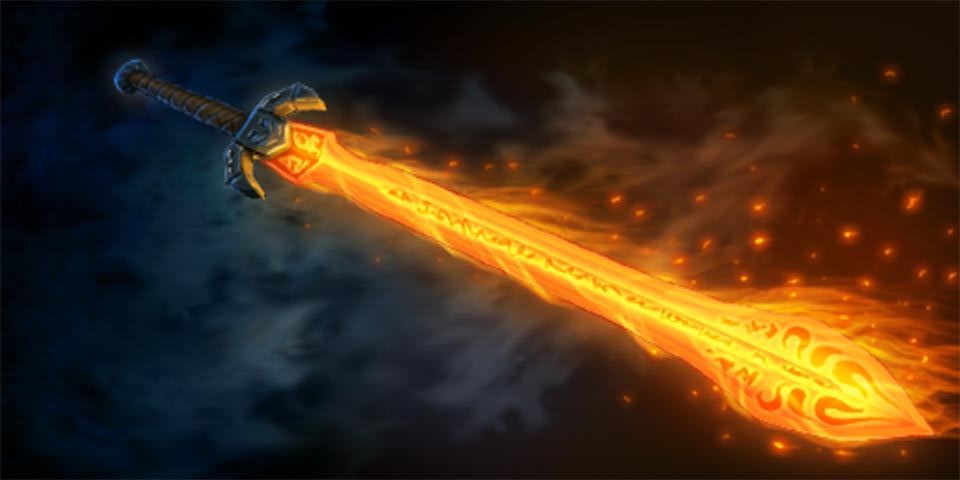A captivating image showcases a magical flaming sword set against a dark and smoky background. The sword, depicted with its hilt at the top left and its blade extending to the bottom right, becomes increasingly engulfed in flames as it reaches the tip. The hilt features a brown-wrapped grip, a rounded stone pommel, and a cross guard resembling double upward horns. The blade itself is vivid with blazing red and bright orange flames that extend beyond the metal, complemented by red sparks flying off and smoke swirling around. The night sky backdrop adds to the mystical ambiance with its fiery clouds and sporadic stars. The smoky effect behind the sword, with visible sparks, further enhances the dramatic and enchanting aesthetic of this weapon of fire.